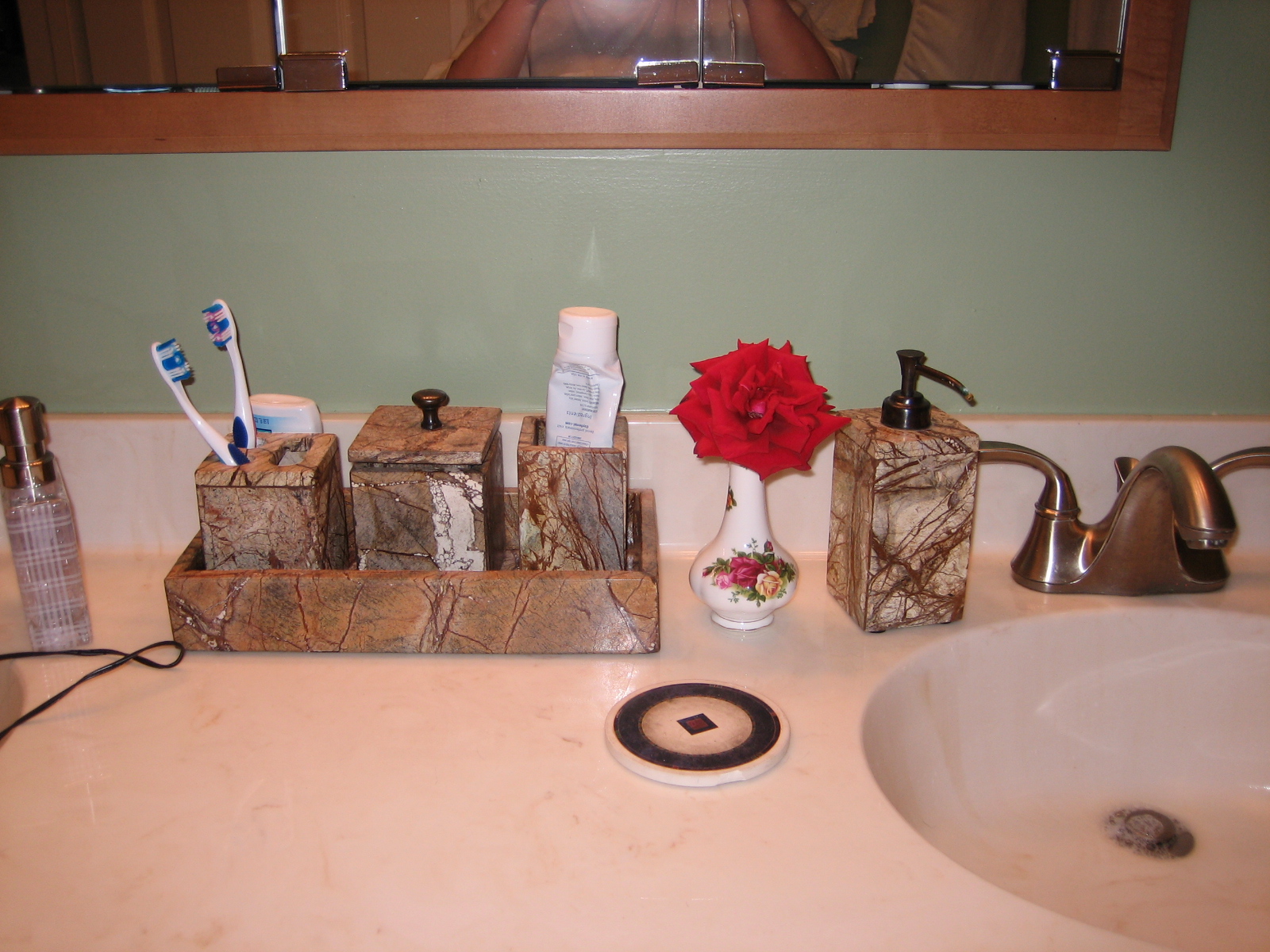The photograph captures a meticulously arranged bathroom countertop, presented in landscape mode. Dominating the upper portion of the image is a wall-mounted medicine cabinet with three mirror-paneled doors, framed in medium-toned maple wood. The reflective surfaces reveal a hint of the photographer, showcasing forearms and part of the chest, suggesting the use of a camera held close to the face.

The wall beneath the mirrored cabinet is painted a calming sage green. The countertop, integrated with a matching backsplash, features a white and cream marbled design, seamlessly incorporating the round sink located on the photo's right side, partly cropped. The sink’s reflective stopper and soap suds hint at recent use, accompanied by a satin nickel faucet.

An assortment of carefully selected items adorns the countertop, enriching the scene with detail and character. Flanking the faucet is a square liquid soap dispenser, resembling moss agate, although likely not made from the actual stone. Adjacent to it stands a delicate bud vase with a white and rose floral design, containing a single, vibrant red rose. Nearby, a round drink coaster with a black border and a central square design adds a functional accent.

A prominent element on the counter is a hefty stone tray, possibly dendritic agate, estimated to be over an inch in height, ten inches in length, and around six inches in width. Inside the tray are coordinated accessories: a toothbrush holder with two toothbrushes, a lidded container with a small knob, and a square tumbler housing a toothpaste tube. To the left, a spritz bottle of perfume with a plaid pattern etched on clear glass and a golden spritz top adds a touch of elegance. An electric cord peeks into the frame, completing the scene with a hint of modern utility.